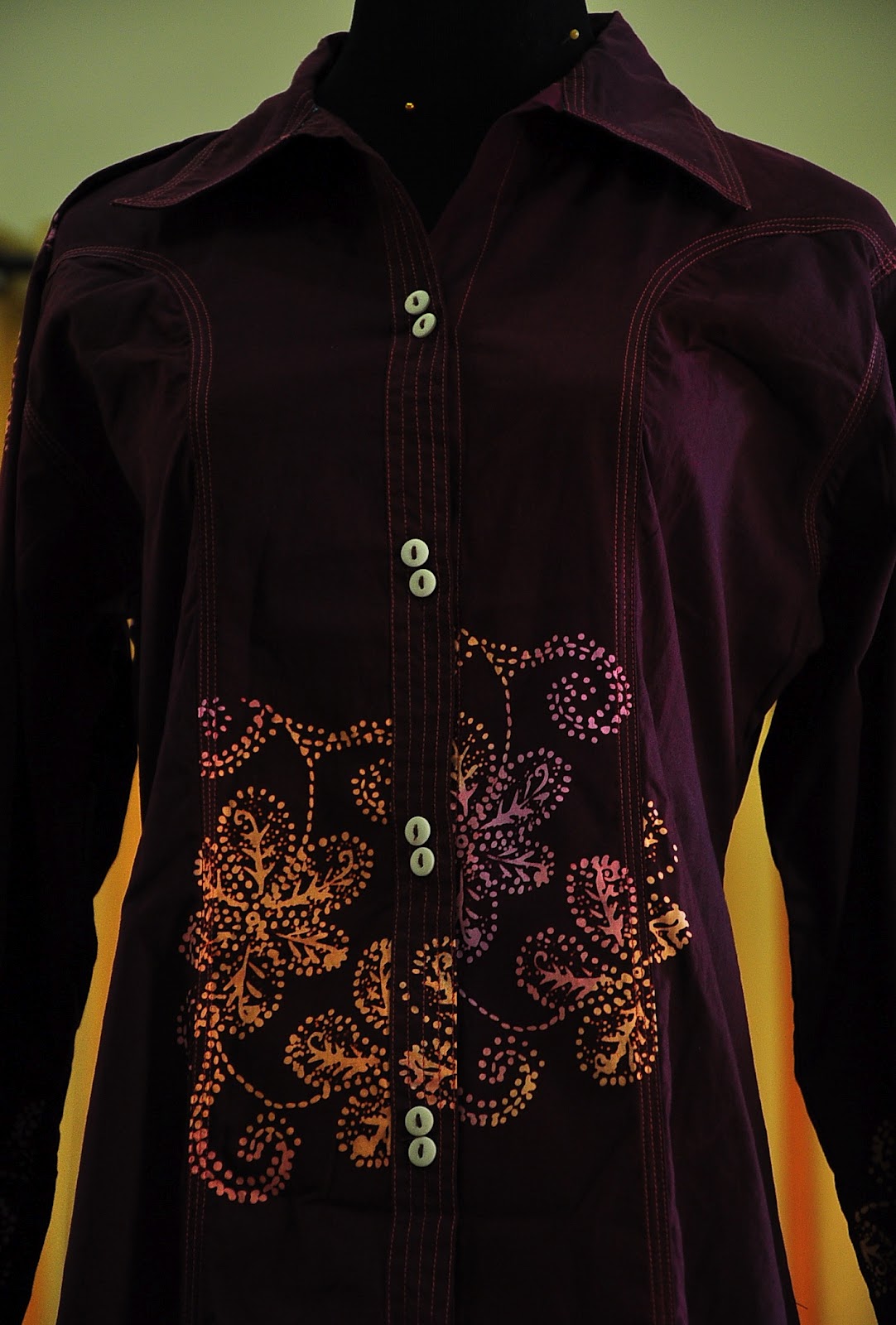This photograph showcases a long-sleeved, velvety shirt presented on the torso of a mannequin. The shirt, which exudes a western country style, features distinctive lines running from the shoulders down to the front and sides, converging into the collar. It's predominantly a very dark purple, though it appears almost maroon or plum, adding to its rich, vivid aesthetic.

The shirt is adorned with a vibrant floral design situated near the stomach area. This design comprises an array of bright colors—pink, light purple, yellow, light red, and orange—created using a pattern of dots that collectively form flowers. The shirt's buttons, which are white with dark thread in the middle, are arranged in pairs, with two buttons placed together followed by a space, repeated down the shirt.

The entire shirt is outlined with a lighter-colored thread that contrasts with its dark base. The setting of the image suggests that it is a product image possibly intended for a clothing advertisement or a website, highlighting the intricate details and textures of this stylish and eye-catching garment.